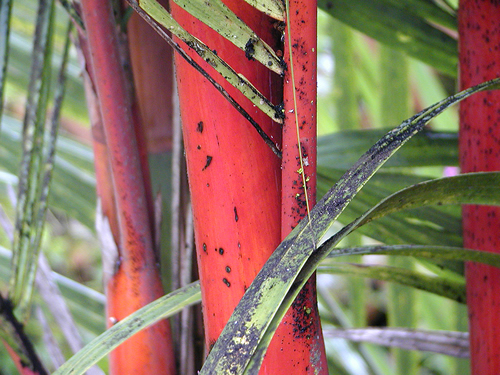This close-up image depicts an intriguing plant with long, slim, narrow leaves that exhibit shades of green and black. The plant, somewhat resembling bamboo in shape, contrasts vividly with a bright red background. The red appears to be some kind of metal object—perhaps a fence or a window frame—though the precise nature is unclear. The scattered arrangement of the green leaves against the striking red backdrop creates a visually compelling scene, highlighting the unique structure and coloration of the plant.